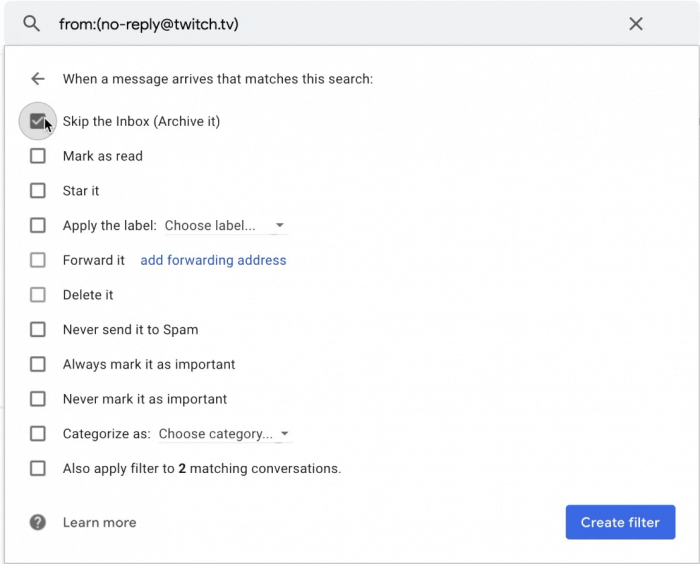This image is a detailed screenshot of an email filter setup within a web-based email client, likely Gmail. The interface has a stark, white background. At the very top, we see a light grey search bar featuring a magnifying glass icon on the left and the text "from:(no-reply@twitch.tv)" within the search bar. On the right end of the search bar, there's an "X" icon for clearing the search criteria.

Below the search bar, a white drop-down menu offers various filter options. The heading of this menu reads "When a message arrives that matches this search," accompanied by a back arrow on the left. This is followed by a series of checkbox options for different actions. The first option, "Skip the Inbox (Archive it)," is currently checked and circled in grey, highlighting its selection. Additional options include "Mark as read," "Star it," "Apply the label," with an associated dropdown menu labeled "Choose label," "Forward it," with another dropdown for "Add forwarding address," "Delete it," "Never send it to Spam," "Always mark it as important," "Never mark it as important," and "Categorize as," accompanied by a dropdown labeled "Choose category."

Towards the bottom of the menu, there is a note on the lower left that says "Also apply filter to 2 matching conversations," giving users an option to retroactively apply the filter. On the bottom right of the interface, there is a blue button labeled "Create filter."